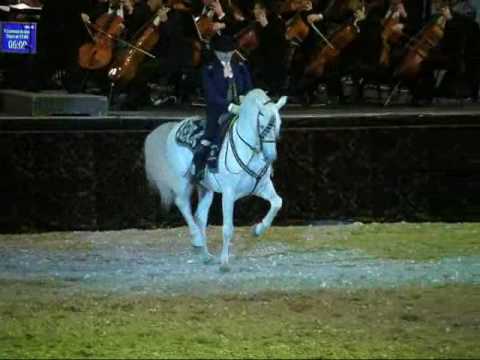In this vibrant and dynamic image, a man, dressed in a navy blue suit and a black hat, is riding a white horse adorned with an intricately decorated blue blanket, or saddle. They appear to be in the center of a grassy ring or arena, likely part of a live performance or circus act. The horse is mid-stride, moving towards the right-hand side of the frame. High above in the background, an orchestra of at least eight violinists and cellists are actively playing their instruments, with their bows moving in unison. This ensemble is arranged on a stage elevated behind the rider. The setting is illuminated by spotlights, emphasizing the live performance aspect. Additionally, a screen with white text is visible in the upper left-hand corner of the image, providing context or announcements related to the show. The entire scene is filled with a sense of motion and anticipation, capturing a theatrical moment of skill and artistry.